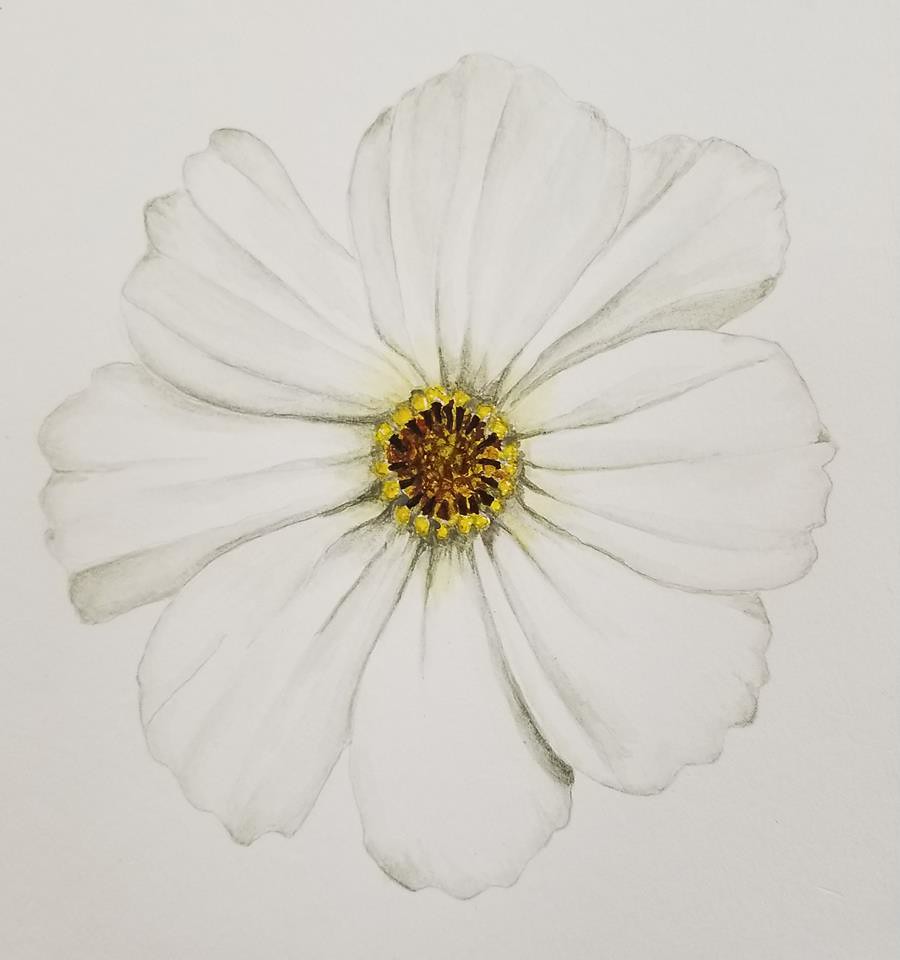The image is a detailed drawing of a flower set against a white background. Predominantly in black and white, the monochromatic theme is broken by a touch of color in the center of the flower. The flower's core consists of bright yellow circular shapes arranged in a larger circle, interspersed with darker circles in shades of brown and tan. Black stripes extend from the yellow circles to the darker central motifs, adding depth and texture. Encircling the center are white petals of varying shapes and sizes, most of which are generously large and wide. Each petal is outlined meticulously in black pencil. The petals feature delicate, light shading, with some exhibiting darker areas mimicking shadows or the slight wilting along their edges, adding a realistic, almost three-dimensional quality to the drawing.